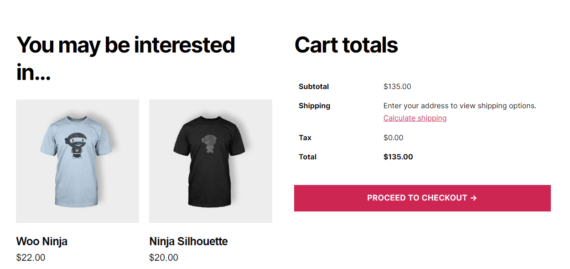The image features a shopping interface with a minimalist design. 

On the left-hand side against a white background, there is black text that reads "You may be interested in...". Below this text are two light gray boxes displaying t-shirts. 

The first box shows a light blue shirt with a navy blue ninja graphic. Beneath this shirt, there is a description that reads "OWO Ninja" with a price tag of $22.00. The second box displays a black short-sleeve shirt featuring a gray ninja silhouette graphic, priced at $20.00.

To the right side of the t-shirts, the cart details are displayed. The header "Cart Totals" is in bold, followed by "Subtotal: $135.00,” and a prompt to "Enter your shipping address to view shipping options," with "Calculate Shipping" highlighted in red and underlined. Below this, "Tax: $0.00" and "Total: $135.00" are noted.

At the bottom right of the screen, there is a prominent red rectangle with white text that reads "Proceed to Checkout" accompanied by a white arrow pointing to the right.